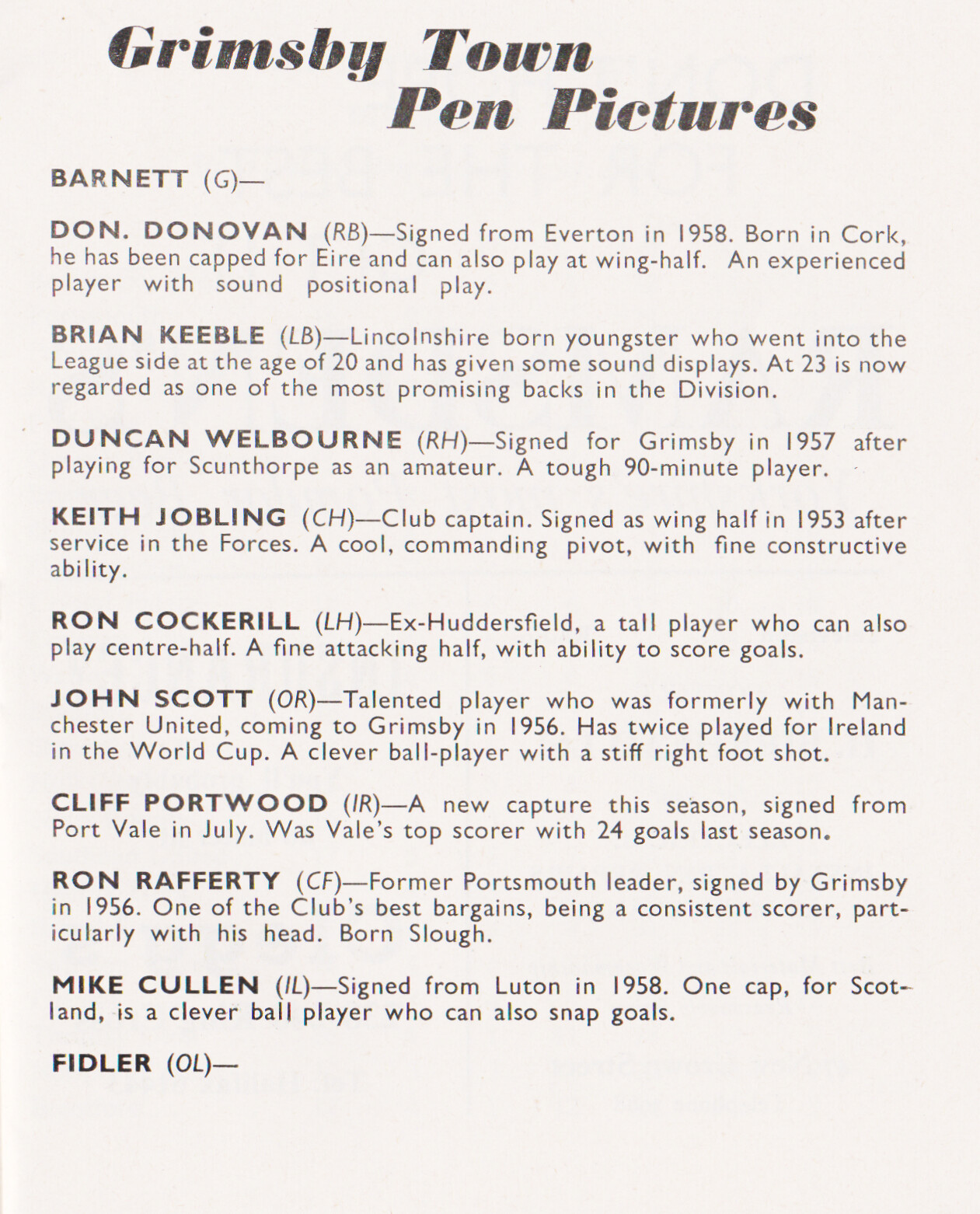The image is a computer-generated picture resembling a playbill or a newspaper clipping with a focus on a soccer team roster. At the very top, in a 70s-era font, it prominently displays the title "Grimsby Town Pen Pictures" in black lettering on a light gray background. The image is horizontally aligned and lists players' names along with their positions and brief descriptions of their careers and abilities.

On the left-hand side, it starts with "Barnett G" followed by details about Don Donovan (RB), who was signed from Everton in 1958, born in Cork, capped for Ireland, and able to play at wing half. Donovan is noted for being an experienced player with sound positional play.

The list continues with:
- **Brian Keeble (LB)**: A Lincolnshire-born youngster who joined the league at 20, known for his promising displays and regarded as one of the best backs at 23.
- **Duncan Welborn (RH)**: Signed for Grimsby in 1957 after playing as an amateur for Scunthorpe, noted as a tough 90-minute player.
- **Keith Jobling (CH)**: The club captain, signed as a wing half in 1953 post-military service, described as a cool and commanding pivot with constructive ability.
- **Ron Cockerill (LH)**: Formerly with Huddersfield, a tall player who can also play center half, recognized for his attacking prowess and goal-scoring ability.
- **John Scott (OR)**: Talented player formerly with Manchester United, joined Grimsby in 1956, twice played for Ireland in the World Cup, known for his clever ball play and strong right foot shot.
- **Cliff Fortwood (IR)**: New recruit for the season, signed from Port Vale where he was the top scorer with 24 goals the previous season.
- **Ron Rafferty (CF)**: Formerly with Portsmouth, joined Grimsby in 1956, considered a bargain and a consistent scorer, particularly with headers.
- **Mike Cullen (IL)**: Signed from Luton in 1958, capped by Scotland, recognized for his clever ball play and goal-scoring ability.
- **Fiddler (OL)**: The list ends with Fiddler, whose position and brief description further establish the document's context regarding sports from the 60s.

The text is a mix of bold uppercase for names and a combination of upper and lower case for the descriptions, providing a vintage feel typical of the era.